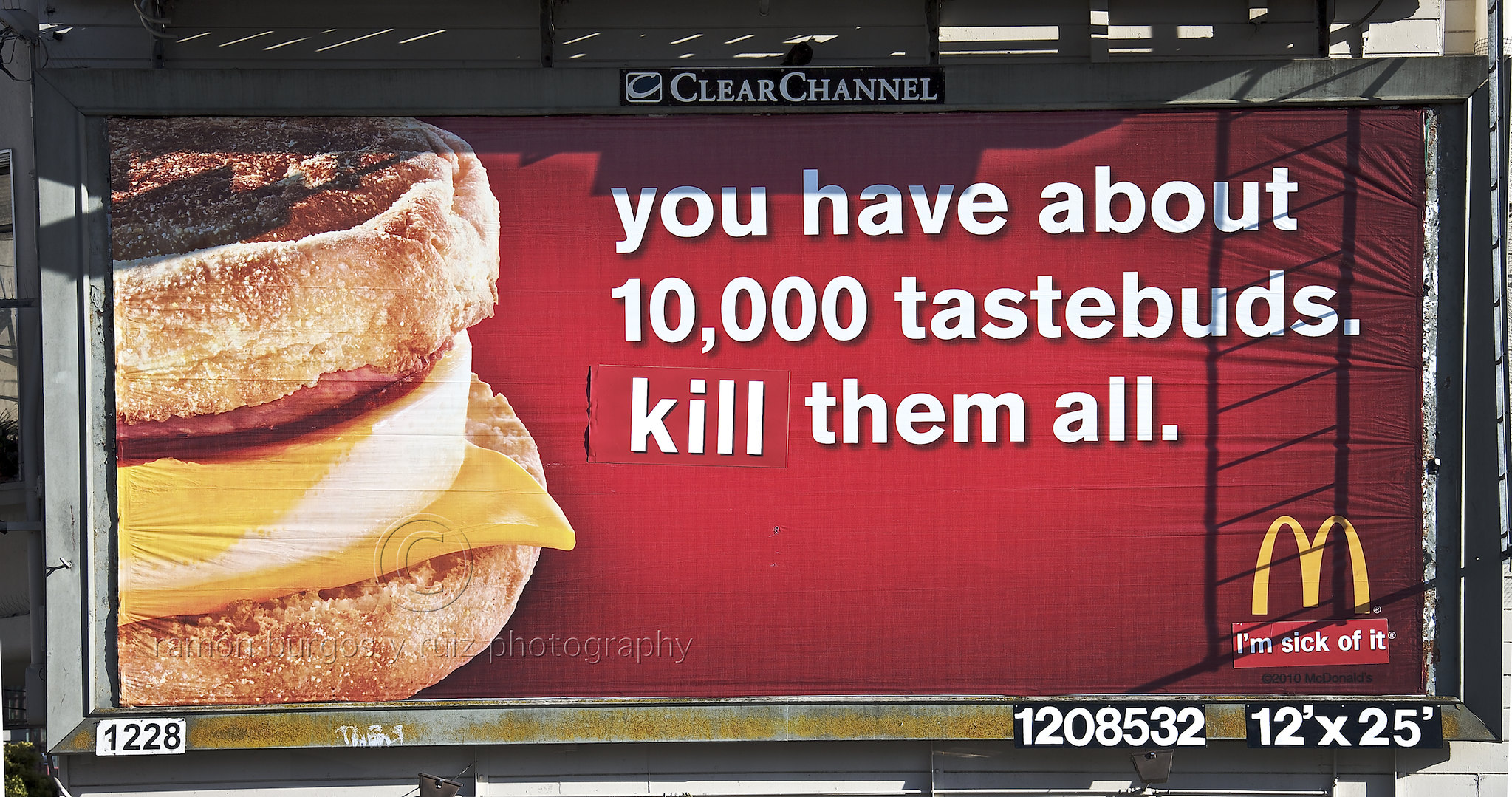In this daytime photograph, the scene is dominated by a large billboard affixed to a beige-colored wall, casting noticeable shadows. The billboard features a vivid red background with an image of an Egg McMuffin on the left side. The text on the billboard provocatively reads, "You have about 10,000 taste buds. Kill them all." The iconic McDonald's "M" logo is positioned in the lower right corner, accompanied by the rebellious statement, "I'm sick of it." At the bottom left corner of the billboard, the watermark "Rui's Photography" is faintly visible, suggesting the source of the image. Additionally, the words "Clear Channel" are displayed in white just above the billboard, indicating the advertising company.